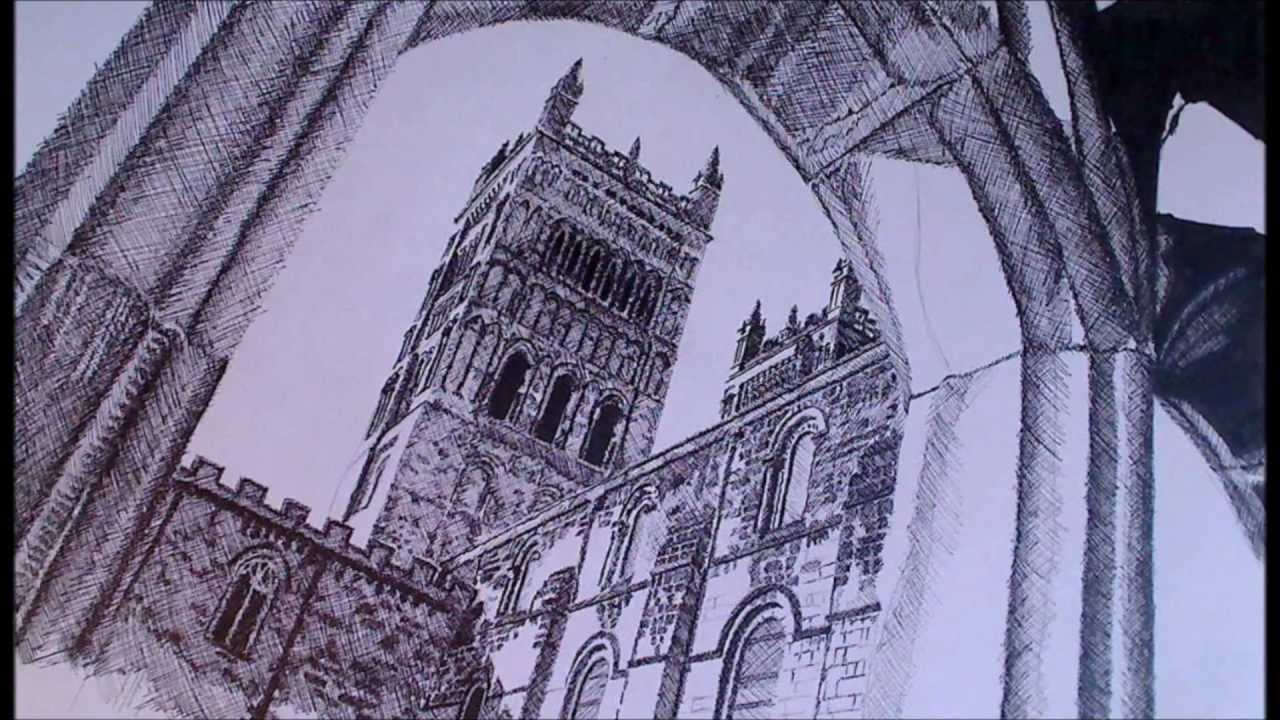The image is a highly detailed, black-and-white drawing or rendering, likely created with pen and ink, pencil, or charcoal. It features an impressive castle structure viewed from a low angle, framed by an arched foreground. The arched entryway leads the eye to a large single-level building that transitions into a massive, vertical tower. The castle is constructed of numerous bricks and incorporates multiple arched windows, giving it an old-fashioned, fanciful appearance. One of the towers features crenelated sections and dark, open archways at the top, with pointy projections at the corners. The scene suggests stone construction throughout. Another tower is barely visible on the right, indicating twin towers. The sky in the background is a light grayish-white, contributing to the monochromatic theme of black, white, and steel gray, textured to highlight the features.